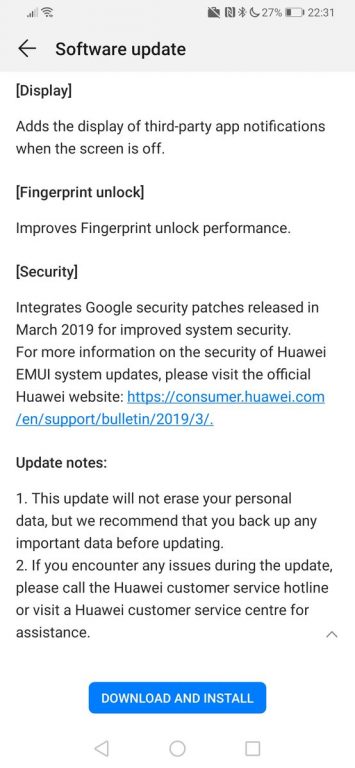This image captures a software update notification screen on a Huawei device. The background is a clear light gray, divided into distinct sections. At the upper section of the screen, there are two rows: the top right corner indicates 22:31 and a 27% battery level. Below this, a black back arrow and bold black text state "Software Update."

The main section of the screen, with a white background, contains detailed update notes. It begins with:

- **Display**: [Includes the display of third-party app notifications when the screen is off.]
- **Fingerprint Unlock**: [Improves fingerprint unlock performance.]
- **Security**: [Integrates Google security patches released in March 2019 for improved system security.]

For more information on the security of Huawei EMUI system updates, a live URL link to the official website is provided in blue text.

The notification continues with "Update Notes," advising that the update will not erase personal data but recommends backing up any important information. If any issues arise, users are directed to contact Huawei customer service.

At the bottom of the screen is a light blue button labeled "Download and Install," which is another main live link alongside the Huawei website URL.